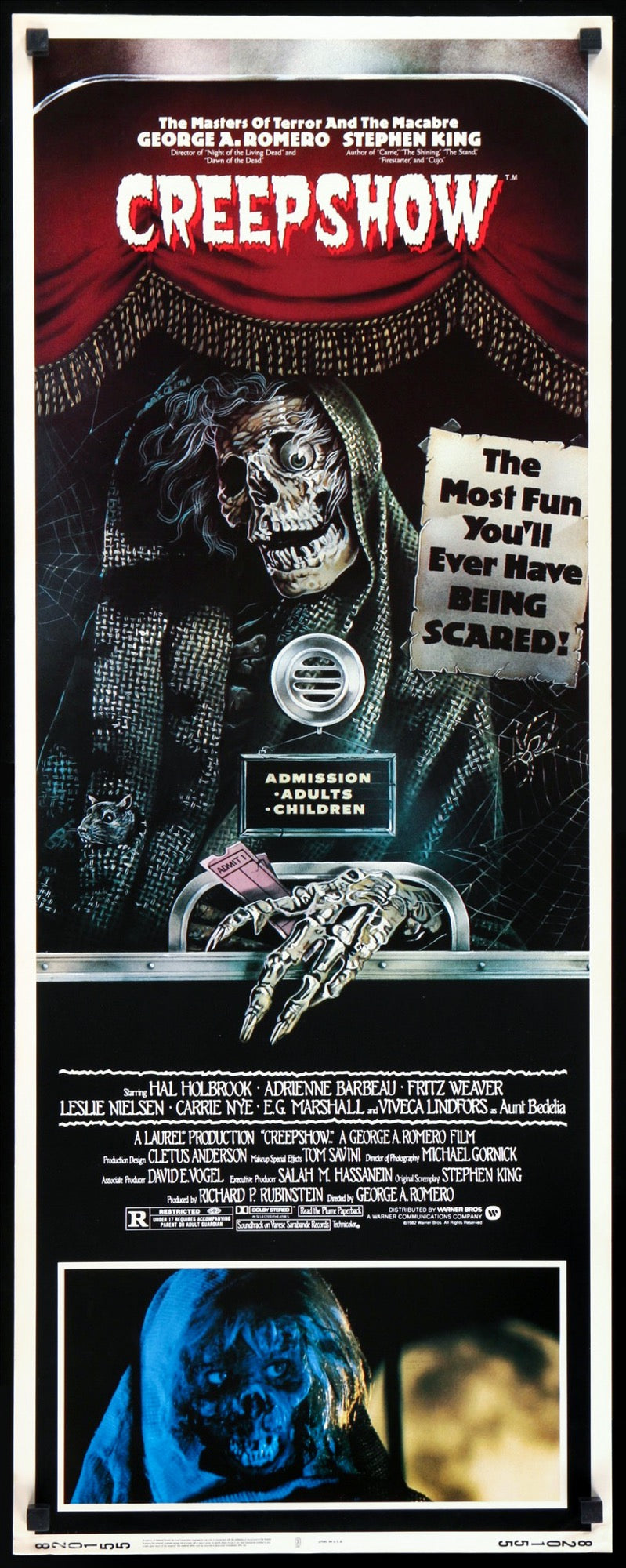The image is a detailed, color movie poster for the film "Creepshow." The poster has an elongated rectangular shape, standing out from typical movie posters. At the top, the banner reads "The Masters of Terror and The Macabre: George A. Romero and Stephen King," emphasizing the collaboration between the renowned horror director and the famous writer. Below this text is the title "Creepshow" written in bold white letters against a red curtain backdrop, similar to those you would find at a theater or ticket booth.

A central feature of the poster is a skeletal figure dressed in a robe, positioned inside a ticket booth. The skeleton leans forward, holding a ticket, giving a haunting welcome to the show. Adjacent to the skeleton, a sign declares, “The Most Fun You’ll Ever Have Being Scared,” highlighting the entertainment value of the horror film. The booth advertises admission prices for adults and children.

The bottom portion showcases a list of notable cast members including Hal Holbrook, Adrian Barbeau, Fritz Weaver, Leslie Nielsen, Carrie Nye, and E.G. Marshall, among others. Below the cast list, another image depicts a skeleton, likely a scene from the film, reinforcing the horror theme. The overall presentation is vivid with ample natural light illuminating every detail, and the atmosphere radiates a blend of terror and excitement fitting for a cinematic experience masterminded by Romero and King.